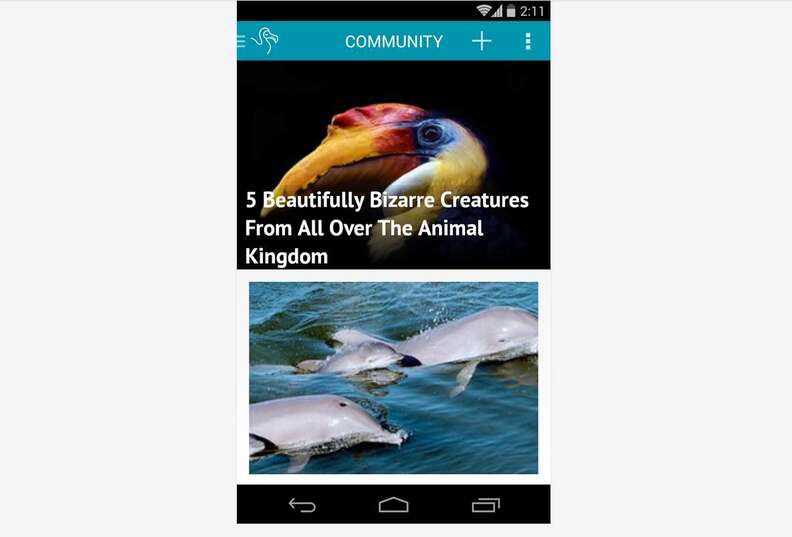The image depicts a printout from an animal website page. At the top, a blue banner displays the word "Community" in white lettering, flanked by a plus sign and three icons—two on each side. Above this, a black banner shows the time "2:11" and three additional icons to its left. Directly below the blue banner, a black background features the title "Five Beautifully Bizarre Creatures from All Over the Animal Kingdom" in white text. Accompanying this title is an illustration of a vibrantly colored, bird-like creature with a striking blue eye and a multi-hued beak displaying shades of red, yellow, gray, and black. Below this, an image of large aquatic creatures, possibly whales or other fish, swims within a deep blue sea that gradates from dark to marine-blue. One fish is detailed enough to reveal its eye marked by a discernible dot.